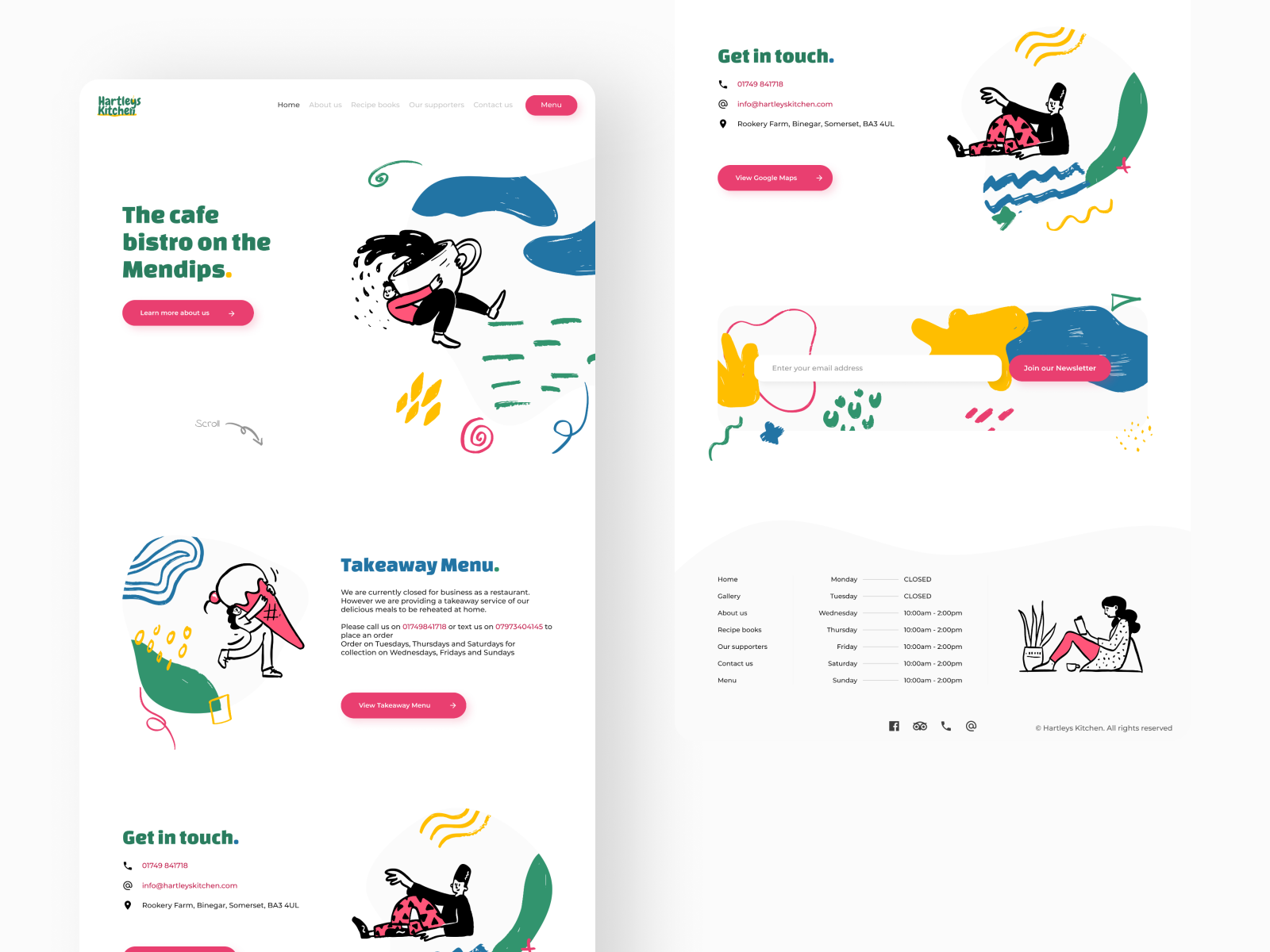The image is divided into two sections, each representing a separate page. 

**Left Page:**
- The background is white.
- The top left reads "Hadley's Kitchen" written in green, underlined with a yellow line. 
- To the right, there are navigational tabs: Home, About Us, Receipt Books, Our Supporters, Contact Us, and a Menu button in pink on the top right.
- The center text reads "The Cafe Bristol on the Mandeeps" in green.
- Below this, there's a pink button labeled "Learn More About Us."
- To the right, a drawing depicts a person wearing a pink jersey, black shorts, and white shoes, holding a large, overflowing white cup with black liquid. The background features artistic designs in blue, green, yellow, and pink.
- Bottom text states: "Takeaway Menu. We are currently closed for business as a restaurant. However, we are providing a takeaway service for our delicious meals to be reheated at home. Please call us on 017-498-41718 or text us on 079-734-04145 to place an order on Tuesday, Thursday, and Saturday for collection on Wednesday, Friday, and Sunday."
- A pink button at the bottom reads "View Takeaway Menu."
- Bottom left text: "Getting in Touch" with contact details: info@hadleyskitchen.com, Rokari Farm, Bineka, Small Somerset.
- Center left features a picture of a person holding an ice cream.

**Right Page:**
- Top text reads "Getting in Touch."
- Below, a pink button labeled "View Cookie Maps."
- Email field labeled "Enter Email Address" with a pink button saying "Join Our Newsletter."
- Bottom left lists: "Home Monday Closed, Galare Tuesday Closed, About Us Wednesday, Receipt Books Thursday, Our Supporters Friday, Contact Us Saturday, Menu Sunday."

This detailed caption captures each element present in both sections vividly.